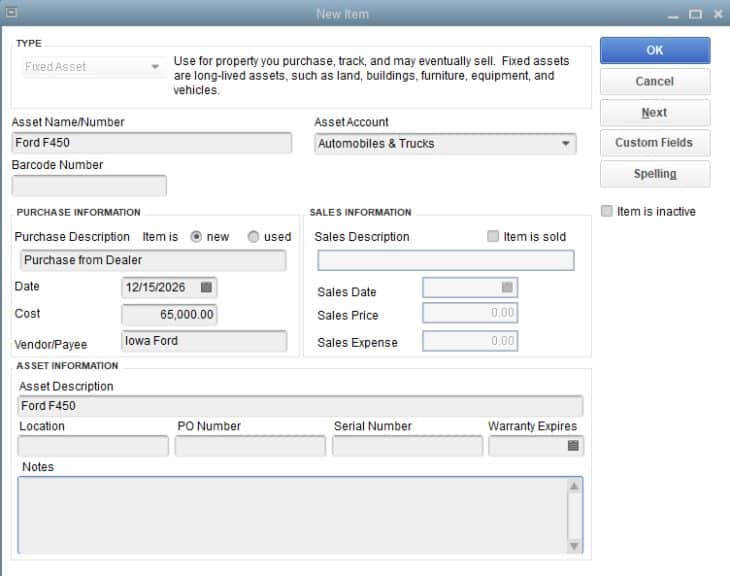The image depicts a form on an electronic device, likely a computer or phone. The interface is structured as follows:

At the top, there is a grayish-blue header with the title "New Item" prominently displayed. On the far right of this header, there is an "X" button for closing the form.

Below the header, the background turns white, and the layout is divided into multiple sections and fields:

1. **Title Section (Upper Left Corner):**
   - The label reads "Top."
   - Directly underneath, there is a dropdown menu labeled "Fixed Asset."
   - An explanatory note to the right of the dropdown states: “Use for property you purchase, track, and may eventually sell. Fixed assets are long-lived assets such as land, buildings, furniture, equipment, and vehicles.”

2. **Action Buttons (Far Right, Vertical Column):**
   - The buttons, listed from top to bottom, are:
     - "OK" (highlighted in blue)
     - "Cancel"
     - "Next"
     - "Custom Fields"
     - "Spelling"

3. **Asset Information (Middle Section):**
   - There is a text field for "Asset Name Number," which has been filled with "Ford F450."
   - Adjacent to this field is another labeled "Asset Account," with "Automobiles and Trucks" typed in.
   - Below these, there is a blank field designated for the "Barcode Number."

4. **Purchase and Sales Information (Lower Section):**
   - The "Purchase Information" subsection includes:
     - "Purchase Description": filled out with "Purchase from dealer."
     - "Purchase Date": "12-15-2026."
     - "Cost": "$65,000."
     - "Vendor": "Iowa Ford."

   - At the very bottom, under "Asset Description," the text "Ford F450" is entered.

This detailed arrangement efficiently captures and organizes crucial information about the fixed asset, adhering to a user-friendly format that facilitates data entry and subsequent modification.